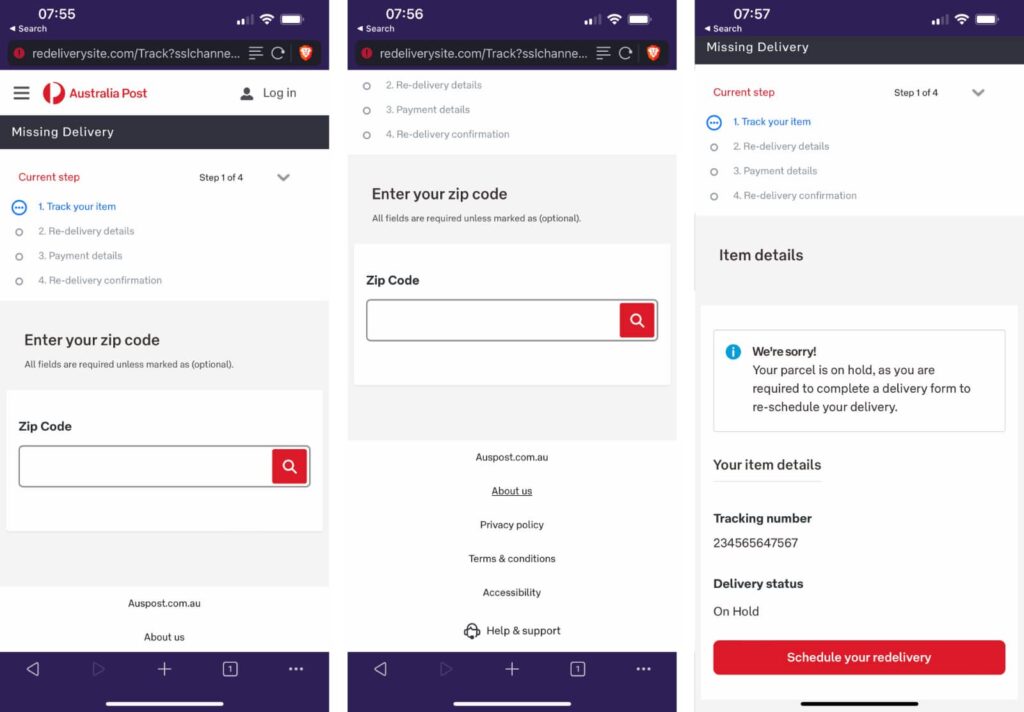The image consists of three screenshots from a mobile device, showcasing different stages of using the Australia Post tracking and redelivery service. Each screenshot displays the following details:

### First Screenshot:
- **Time Displayed:** 7:55 AM
- **Upper-right Icons:** Wi-Fi strength and battery status
- **Search Bar:** White font on a black line with a red dot beneath it
- **URL Displayed:** `redeliverysite.com/track?SSLchannel`
- **Menu Icons:** Three lines indicating a menu, and a refresh button
- **Top Menu:**
  - **Australia Post Logo** with "Australia Post" text
  - Three lines icon next to it for another menu
  - **Login Icon:** Head and shoulders of a person with "Log In" text beside it

### Second Screenshot:
- **Time Displayed:** 7:56 AM
- **Same Upper-right Icons:** Wi-Fi strength and battery status
- **Current Page Title:** "Missing Delivery," in white lettering on a black box
- **Tracking Details:**
  - **Current Step:** Step 1 of 4, "Track Your Item" in blue
  - Next steps: 
    1. Redeliver Details
    2. Payment Details
    3. Redeliver Confirmation
- **Form Instructions:** All fields required unless marked as optional
- **Zip Code Field:**
  - Enter your zip code, with a red search key beside it
- **Website Footer Information:**
  - `autopost.com.au`
  - Menu options: "About Us," "Privacy Policy," "Terms and Conditions," "Accessibility," "Help and Support"

### Third Screenshot:
- **Time Displayed:** 7:57 AM
- **Notice Detail:**
  - Blue circle with a white 'i' icon for information
  - **Message:** "We're sorry, your parcel is on hold as you're required to complete a delivery form to reschedule your delivery."
- **Parcel Details:**
  - Tracking Number: 2345656647567
  - Delivery Status: "On Hold"
- **Action Button:** Red box with "Schedule Your Redelivery" in white lettering
- **Footer:** Black line below the action button, consistent with the design in the other images

The images depict a user navigating through Australia Post's mobile interface to track and reschedule the delivery of a parcel, showing time progresses during their interaction.